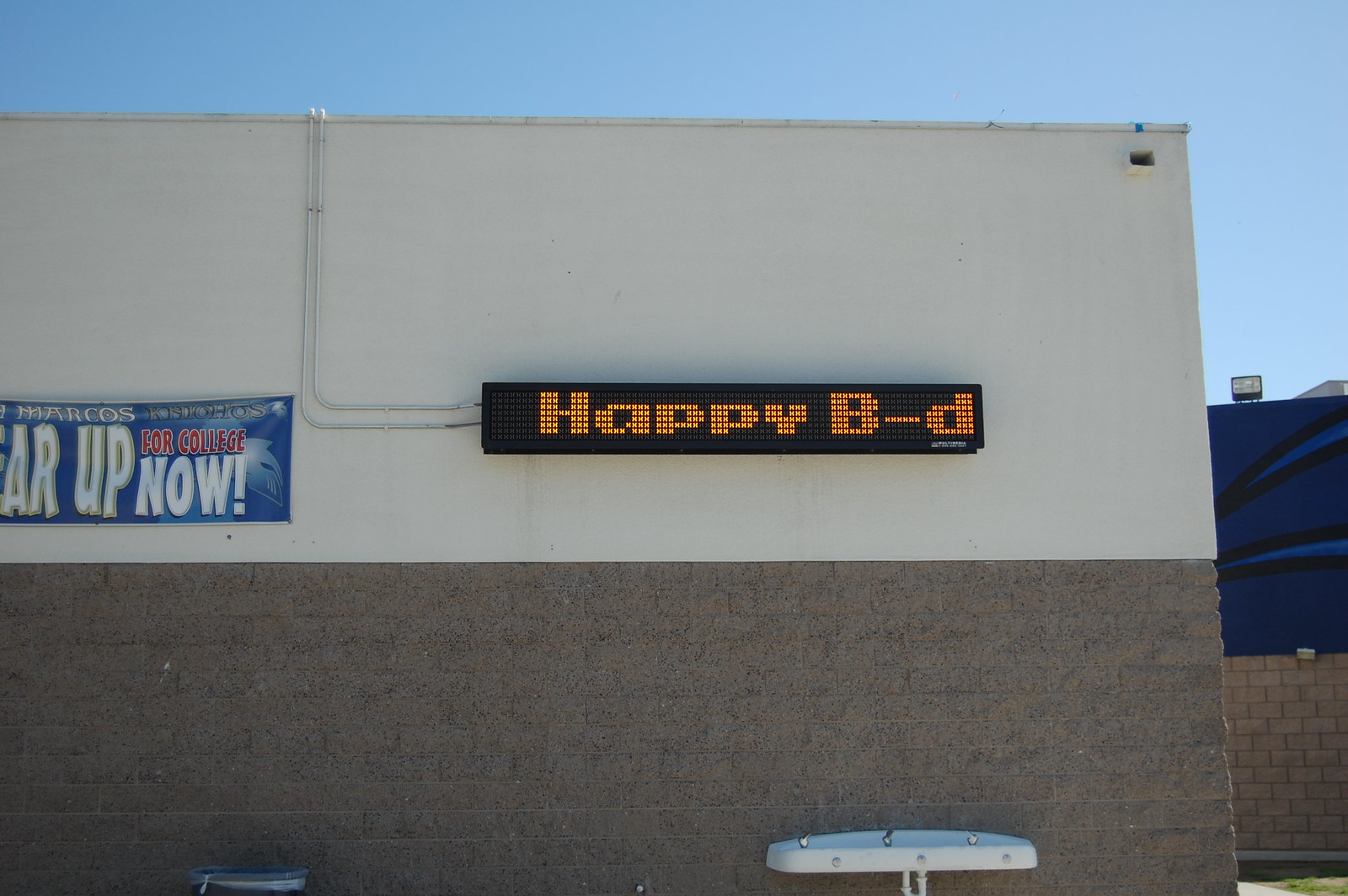The photograph showcases the side of a building under a clear, bright sunny sky. The building itself features a combination of white paint and brown brick that starts from the middle and goes downwards. An electric black sign is prominently displayed, glowing with cheerful yellow text that reads "Happy B-D." Adjacent to this sign is a vibrant blue mural painted on the building’s side, incorporating shades of black and light blue in its design.

Additionally, next to this main building, another structure might be present, hinting at an urban setting with multiple edifices. A blue banner with white lettering is also visible, adorned with red text that states, "For college." The banner further includes a motivational phrase, "Gear up now," with the name "Marcos" positioned at the top. This scene captures a moment on a lively, sunny day, enhancing the vivid colors and festive atmosphere.